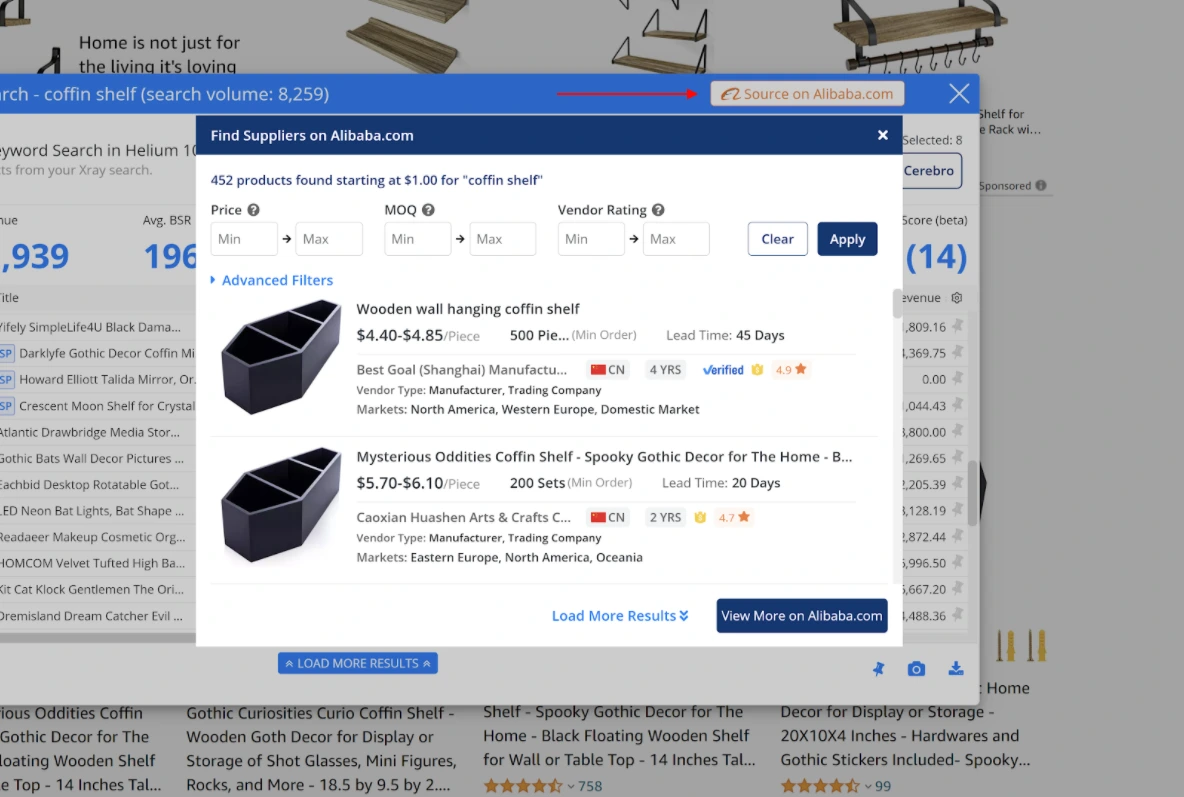This image, sourced from Alibaba.com, showcases a search for "coffin shelf" conducted by a user. The user has discovered 452 different products, with prices starting at $1. In the background, further search results display a search volume of 8,259 for similar products on Alibaba. The image hints at additional browsing activities on another e-commerce site, likely Amazon, where the user appears to be exploring gothic home decor options, including wooden wall shelves and gothic stickers. The overall context suggests that the user is meticulously comparing multiple platforms to find the perfect black coffin-shaped shelves for their gothic-themed decor.